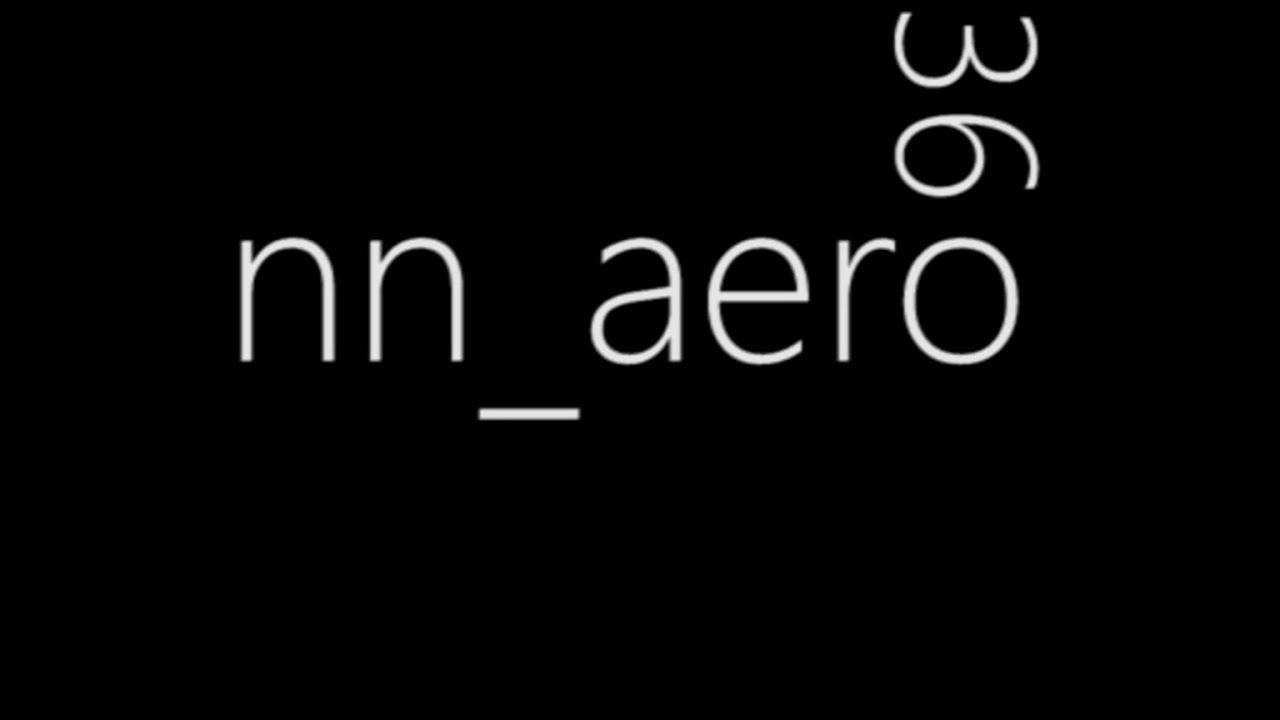The image features a pitch-black background with crisp, clean white lowercase letters arranged horizontally across the midsection: ‘n’, ‘n’, an underscore, ‘a’, ‘e’, ‘r’, ‘o’. Just above the letter ‘o’, vertically oriented, are the numbers ‘3’ and ‘6’, with ‘3’ positioned above ‘6’. The underscore sits a little below the center, more to the left, separating the pair of 'n's from the sequence 'a', 'e', 'r', 'o'. The entire composition seems to bisect the image horizontally, with the underscore providing a distinct separation under the letters. The corners and most of the bottom part of the image remain completely black.